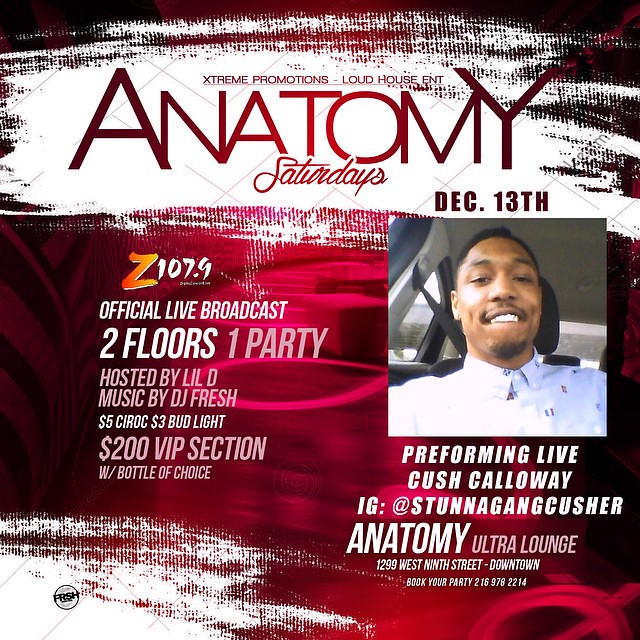This is a detailed advertisement poster for a nightclub event. The background features a blend of burgundy and red hues accented with splashes of white. The focal point on the right-hand side is a smiling African American man in a white shirt, identified as Kush Calloway, who will be performing live. His Instagram handle is @stunnagangkusha. Above his image, the date "December 13th" is prominently displayed. Below him, details such as "Performing Live," "Kush Calloway," and the venue "Anatomy Ultra Lounge" at "1299 West 9th Street, Downtown" are noted, along with a booking phone number: 216-978-2214.

At the very top of the flyer, "Extreme Promotions" and "Loud House ENT" are noted, along with "Anatomy Saturdays" rendered in bold red font with 'Anatomy' in block letters and 'Saturdays' in cursive. On the left-hand side of the poster, additional event details are listed: "Z107.9 Official Live Broadcast", "Two Floors, One Party," hosted by Lil D with music by DJ Fresh, featuring $5 Ciroc, $3 Bud Light, and a $200 VIP section with a bottle of choice. The flyer also features stylistic white paint streaks and blurred lights to enhance the vibrant atmosphere.